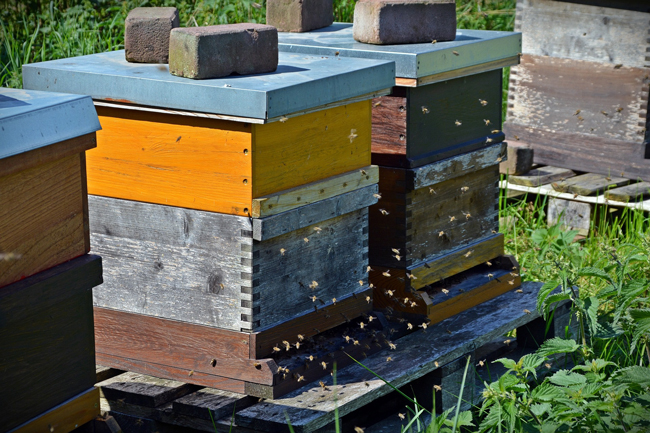On a bright, sunny day, an array of colorful beehives sits quietly amidst a grassy, weedy area, casting distinct shadows under the radiant sunshine. The image prominently features four beehives, two of which are fully visible and actively buzzing with bees. These beehives, resting on old, weathered pallets, exhibit a variety of wood finishes—ranging from weathered, reddish-brown to unfinished, untreated tones. The hives are capped with metal lids, each securely held down by two bricks. The closest hive to the camera has an orange top half and untreated wood at the bottom, while another nearby hive showcases dark brown wood. The scene captures the activity of bees diligently flying around, framed by the green grasses and tiny weeds that grow abundantly around their colorful domiciles.